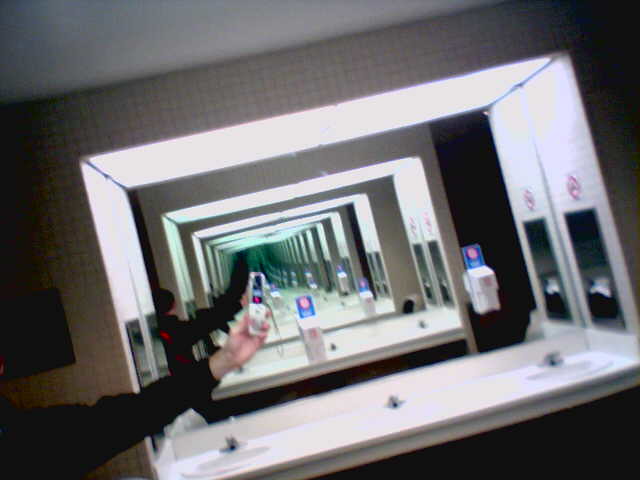The photograph, though somewhat blurry and slightly off-kilter, captures a public restroom with a repetitive, infinite reflection effect. The image centers on a row of three white porcelain sinks, each equipped with silver metal faucets and numerous soap dispensers, set against a wide mirror. The restroom is equipped with multiple dispensers for soap and paper towels, visible on both the left and right sides. A person, dressed in a blue and red sweater, stands centrally holding up an unknown device, likely a phone, adding to the infinite mirror illusion as his reflection echoes endlessly into the distance. The restroom also features a trash can with a white liner slightly exposed, and a no-smoking sign is visible in the frame. This recursive, mirrored effect creates an impression of an endless passageway of sinks and dispensers, enhancing the unique and slightly surreal quality of the photograph.